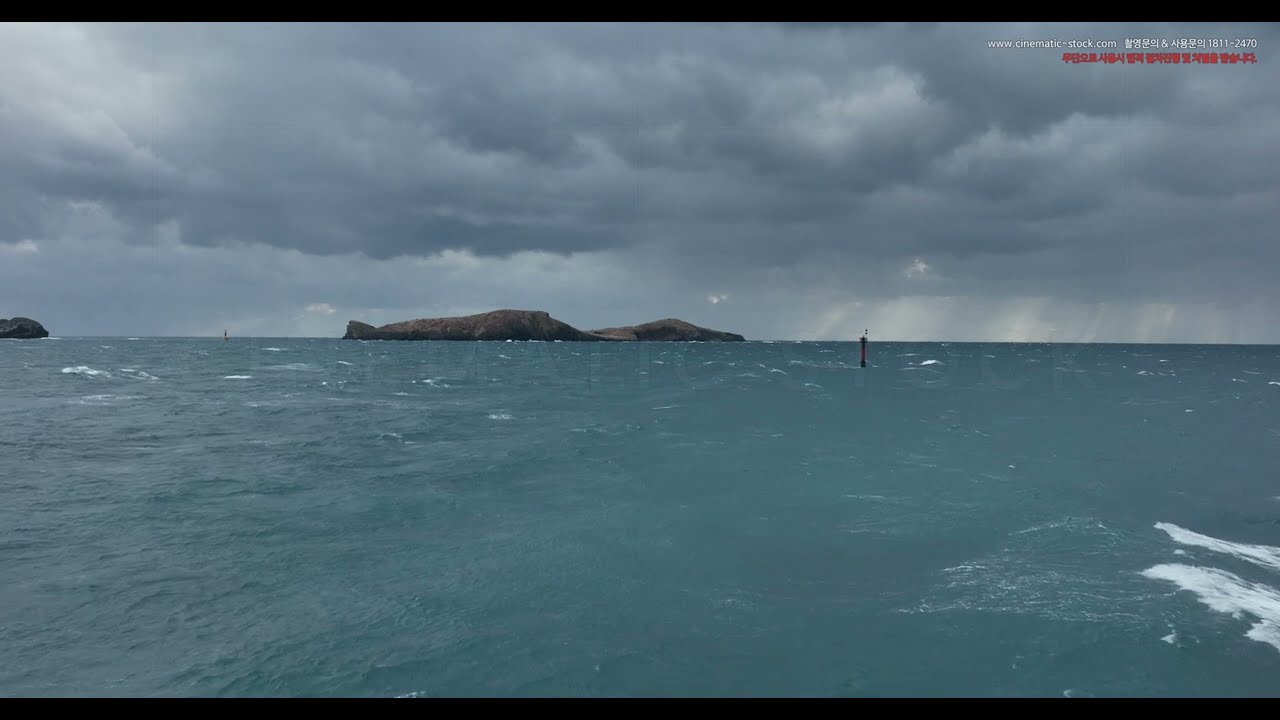The image depicts a scenic ocean view with light bluish-green water, slightly choppy with small crashing waves creating white froth. The sky is overcast with heavy gray clouds, indicative of stormy weather. In the center background, there are prominent rocky structures that resemble a hilly island, while to the left a smaller rock formation can be seen. The serene yet tumultuous scene is dotted with a few buoys floating in the water. Rays of light manage to peek through the clouds in the upper right-hand corner. Faint text in the upper right-hand corner of the image reads "www.cinematic-doc.com," accompanied by additional text in either Korean or Japanese below it. The color palette is dominated by grays and blues, with hints of brown from the rocky islands, capturing the prelude to a storm.